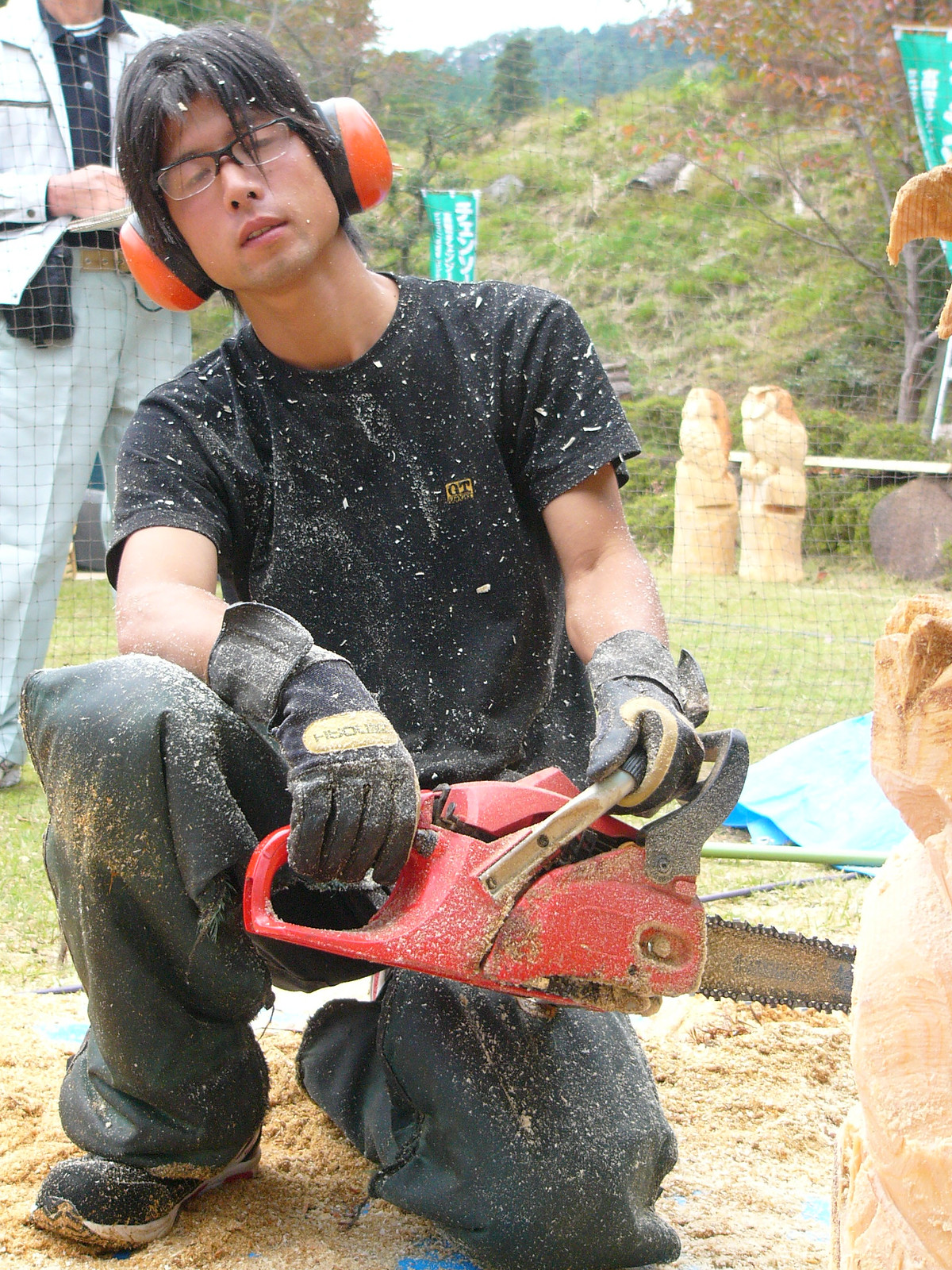In this detailed image, a man is kneeling on one knee in a fenced area, engrossed in carving a wooden sculpture with a red chainsaw, accentuated by its black handle and facing the right. His attire includes black or gray cargo pants, a black shirt with the word "QT" visible, gloves, orange and black earmuffs for industrial protection, and protective glasses. Sawdust covers his work clothes and the ground around him, which is either dirt or a blue tarp scattered with debris. The man's longer, shaggy hair and relaxed demeanor suggest a moment of pause or a shift in his sculpting action. Behind the fenced area to the left, a man stands, possibly judging the scene with a clipboard or papers, dressed in beige or yellow pants and either a black undershirt or a blue shirt. The background reveals a hillside dotted with rocks and plants, and several wooden sculptures, resembling owls carved from logs, indicating completed works. The overall setting might imply a competitive or formal event focused on wood carving.